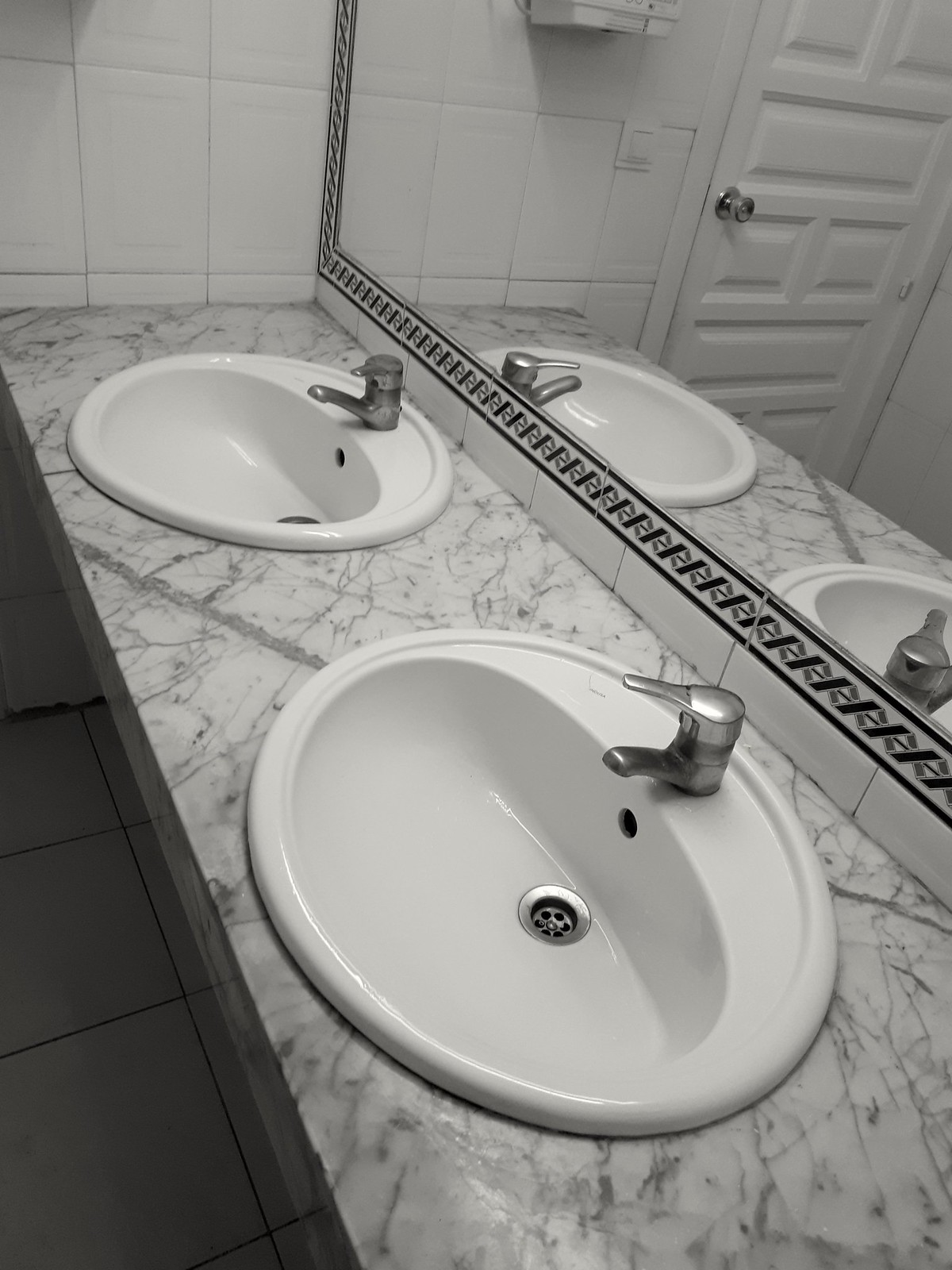This image captures a bathroom vanity, most likely situated in a public or commercial restroom. The vanity features a marble countertop with a typical white background and gray marbling. It houses two standardized white sinks, each equipped with a single-handle faucet. The faucets have long handles positioned above the spout. Behind the vanity stretches a large mirror framed by a black and white tile pattern that coordinates with the wall tile. The wall tiles are rectangular, while the floor tiles are large and square-shaped. Reflecting in the mirror, you can glimpse a white door with a doorknob, suggesting it leads to another part of the restroom. Also visible in the reflection is the bottom part of what appears to be a paper towel dispenser or similar fixture on the wall near the door. The overall color scheme and presence of standardized fixtures and an industrial light switch suggest this is likely a public restroom, possibly in a restaurant.